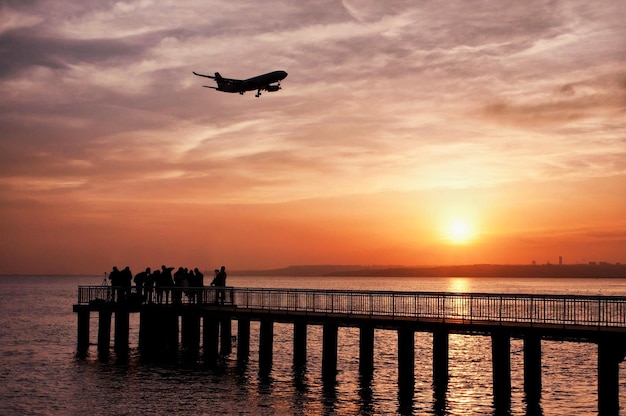This photograph captures a visually striking sunset scene on the ocean, dominated by a long pier extending into the water, supported by multiple poles. At the end of the pier, a group of people is gathered, standing, talking, and watching the sun as it sets. The sky is painted in hues of orange and yellow near the horizon, transitioning to darker shades of blue as it ascends. Silhouetted against this backdrop are the pier, the people, and a large passenger plane flying above, seemingly on a landing approach. A strip of land can be seen far beyond the water, also silhouetted against the colorful sky. The water reflects the sunlight, with brighter reflections on the right side and diminishing towards the left. The scene is alive with details, including the presence of clouds, one person setting up a tripod, and the serene yet dynamic interplay of light and shadow. The sunset's orange and yellow glow enhances the dramatic contrasts, making the people, pier, and airplane appear as striking black silhouettes against the vivid sky.